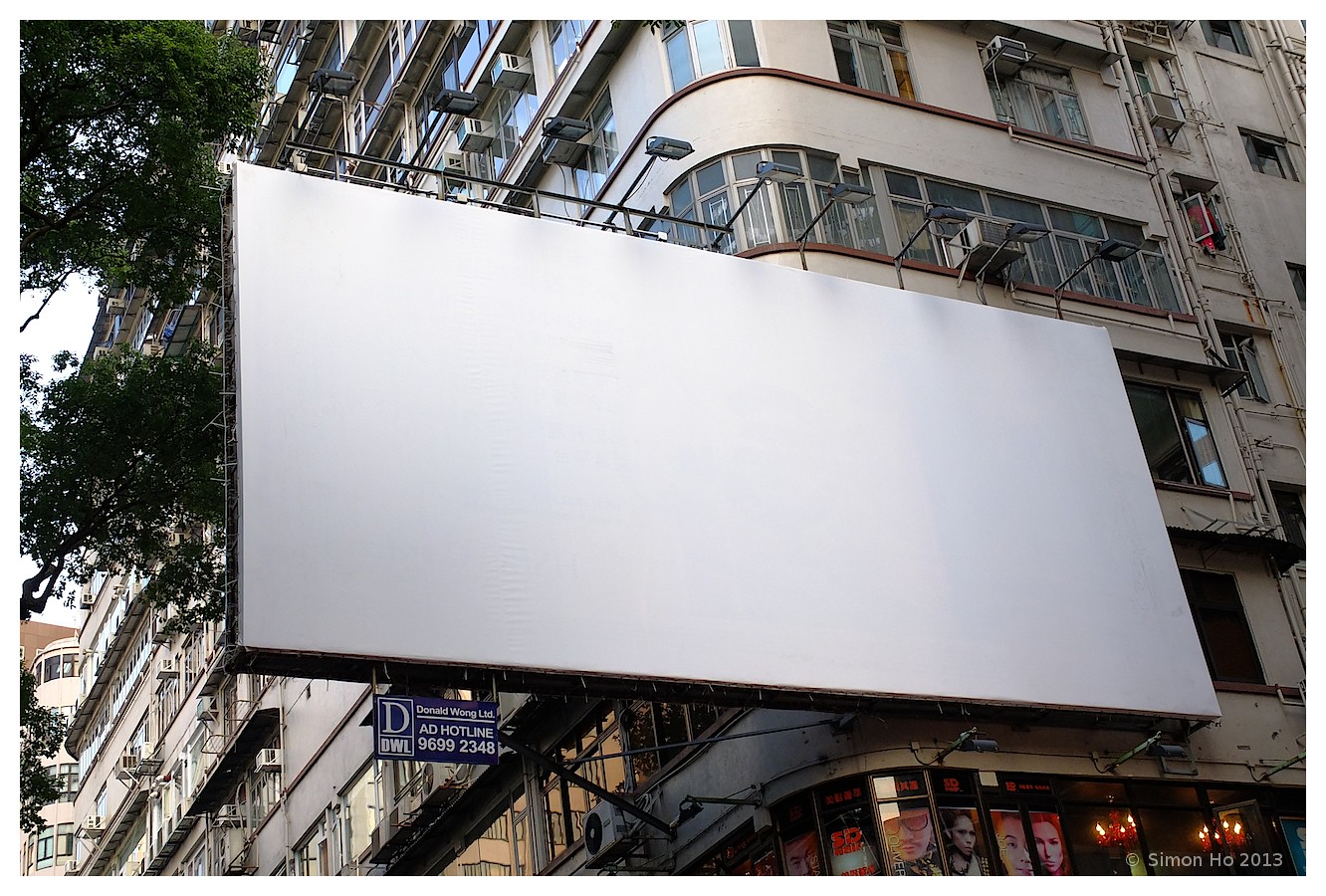On a cloudy, overcast day, an empty white billboard is prominently displayed in this photograph, attached to the corner of an old, cream-colored building with rounded edges. Heavy metal brackets hold the billboard in place, and a row of lights at its top lie dormant against the daylight. Numerous windows punctuate the building's facade, some of which are equipped with air conditioning units. The ground floor appears to house a retail business, possibly a salon or clothing store, as indicated by the illuminated interior and various posters in the windows. Adjacent to the building is a large tree, its top branches and leaves visible. The photo is credited to "Simon Ho, 2013," as indicated in the bottom right corner.